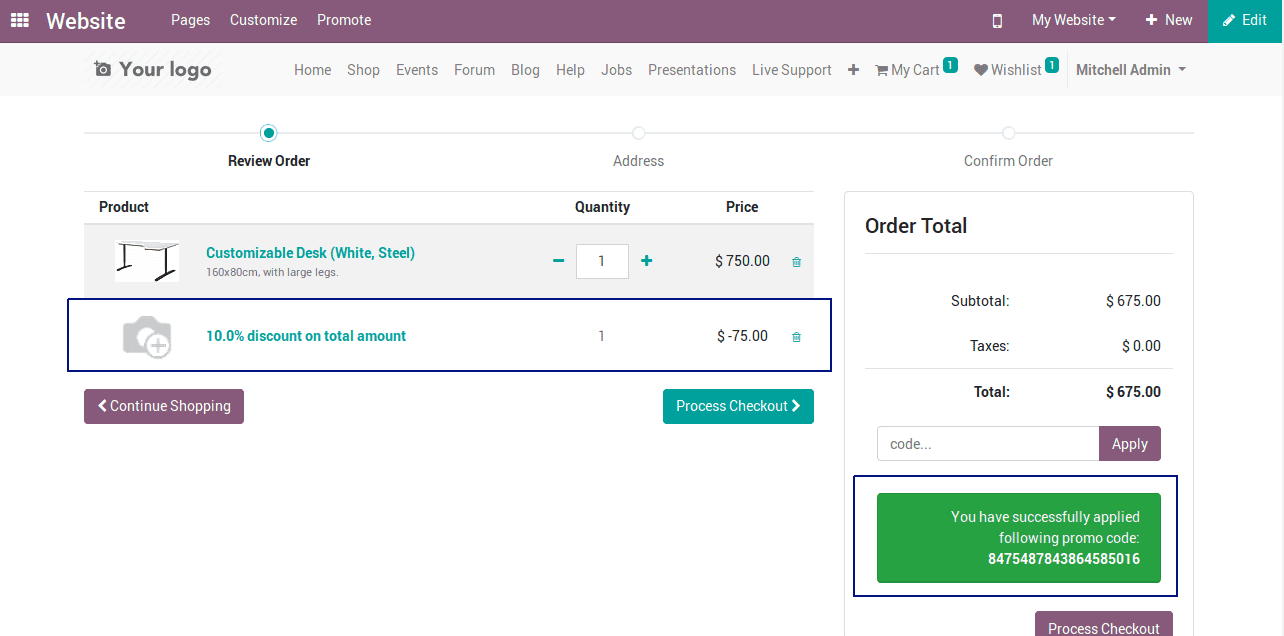The image is a horizontally rectangular screenshot of a website's order review page. At the very top, there's a thin, purple horizontal banner. On the top left, the banner displays the website’s main navigation options: "Website," followed by "Options," "Pages," "Customize," and "Promote." To the right side of the banner, it shows "My Website," "Add New," and a green "Edit" button. 

Below this banner, the background is predominantly white. The website's logo is positioned prominently. Adjacent to the logo is a series of navigation links: "Home," "Shop," "Events," "Forum," "Blog," "Help," "Jobs," "Presentation," "Live Support," "My Cart," "Wish List," and "Mitchell Admin," which seems to indicate the logged-in user's account information.

The main content of the page is the order review section. It begins with a product listing for a customizable white steel desk priced at $750. A discount of 10%, amounts to a $75 deduction from the total price. Below the product details and discount information, there are two actionable buttons: a "Continue Shopping" button on the left and a "Process Checkout" button on the right.

To the far right of these buttons, a summary box details the order total. It lists the subtotal as $675, with taxes shown as $0, and confirms the final total as $675.